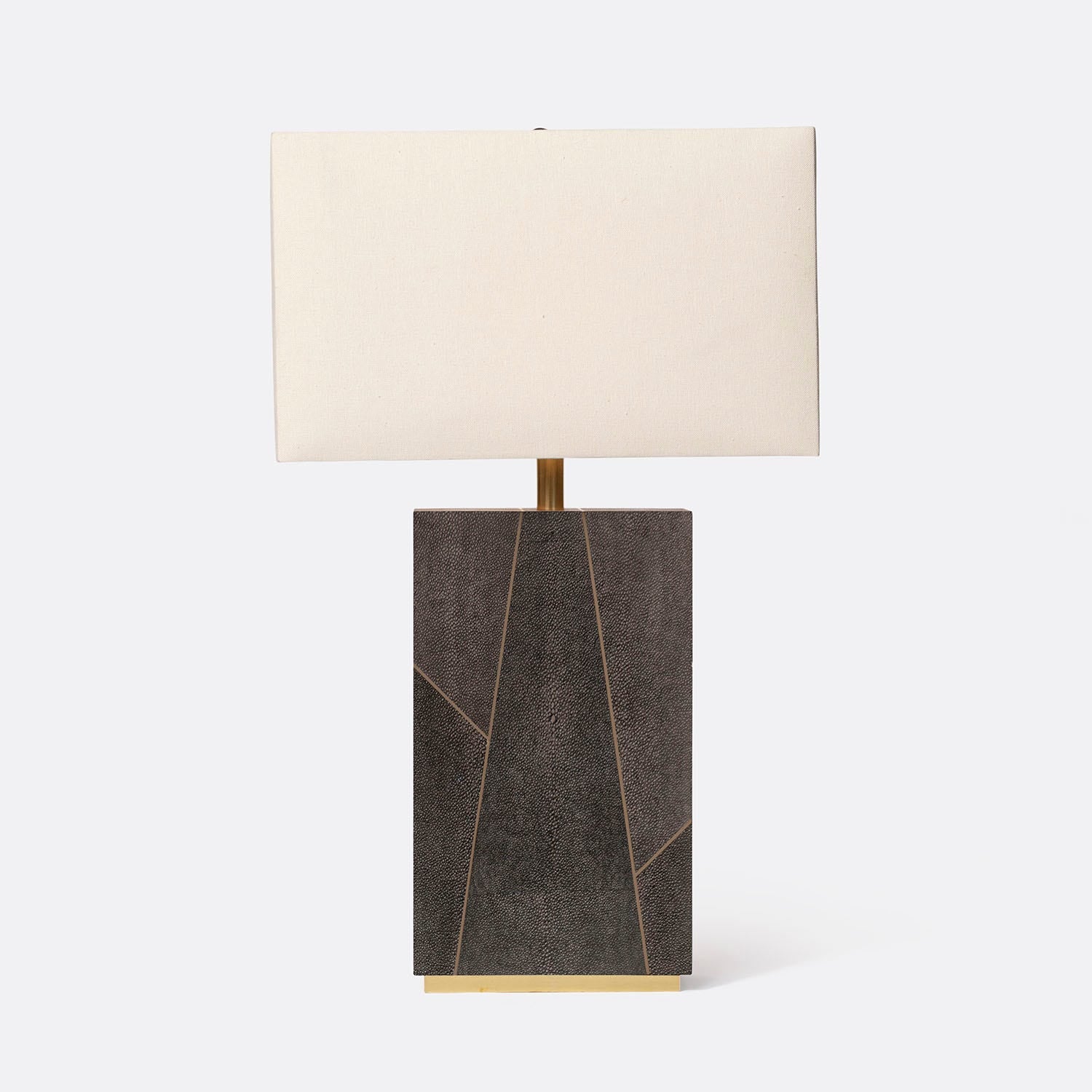The image displays a unique lamp designed to resemble a picket sign. The lamp features a white, blank rectangular sign acting as the lampshade, mounted on a sturdy wooden stick, which holds the lightbulb. The wooden stick extends from a decorative podium that has a black base with an intricate geometric pattern of rectangular shapes, highlighted by fine golden lines. The podium is adorned with purplish speckles and rests on a golden base. The entire structure is set against a light blue background, enhancing the contrast and making the white lampshade stand out prominently.